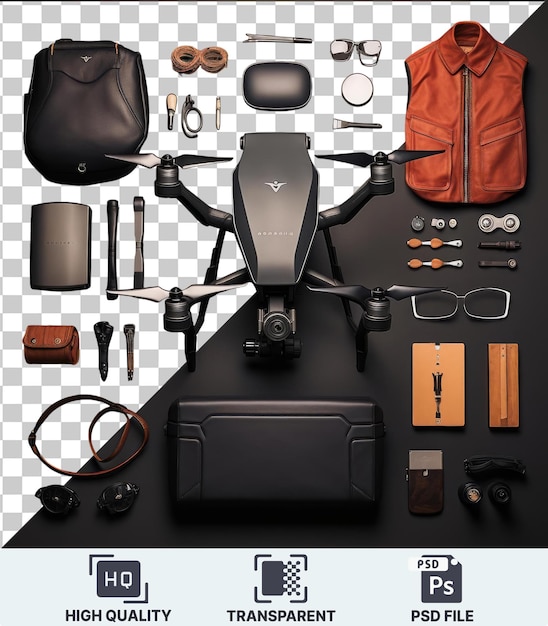The image showcases a transparent PSD file featuring high-quality drone equipment and travel accessories against a checker-patterned and black background. Central to the photograph is a quadcopter drone, crafted from black and gray sheened material, equipped with a camera at the front. Surrounding the drone are various accessories and travel essentials. To the left, there are bags, clutches, and leather bands designed for easy handling. Above the drone are additional items, including glasses, cases, and mirrors. On the right side, a red leather jacket vest and more accessories are displayed. The bottom of the image features a gray border with a clear label and icons that state "HQ High Quality," "Transparent," and "PSD File."